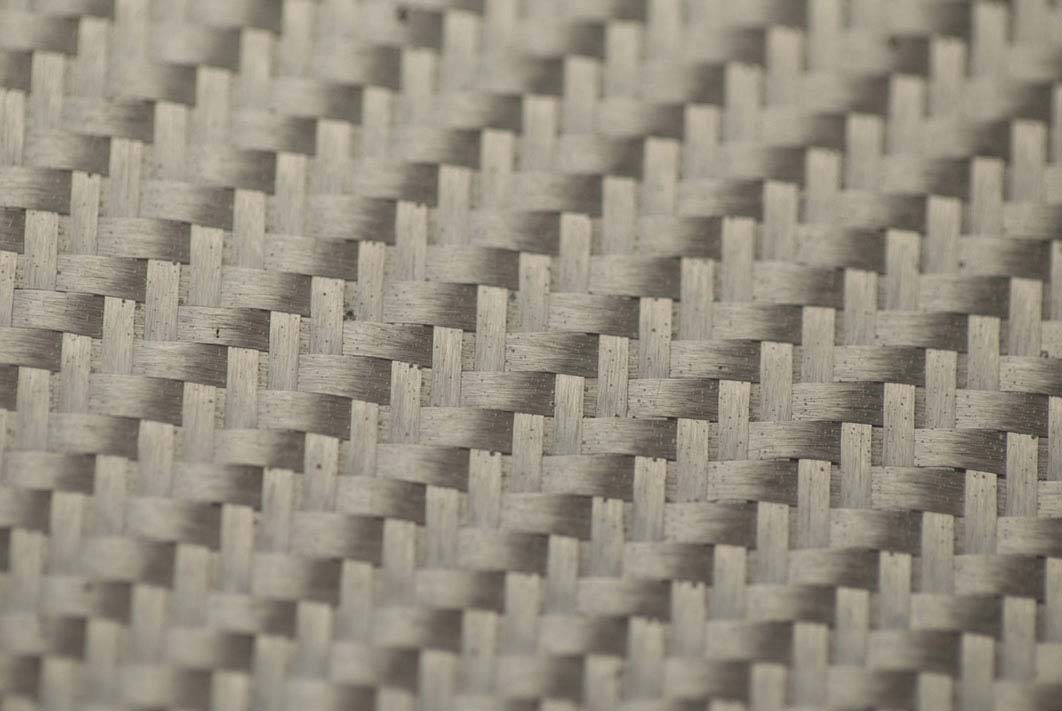This image showcases a highly detailed, close-up view of a tan-colored woven item, resembling the texture often seen in wicker baskets, placemats, or grass rugs. The woven pattern forms an offset lattice or diagonal L shape, with horizontal strands interlacing with vertical hoops. The central part of the image is in sharp focus, while the edges blur slightly, emphasizing the intricate weave of the material. The predominant color is a natural tan, evoking the look of traditional wicker or fabric used in patio furniture.